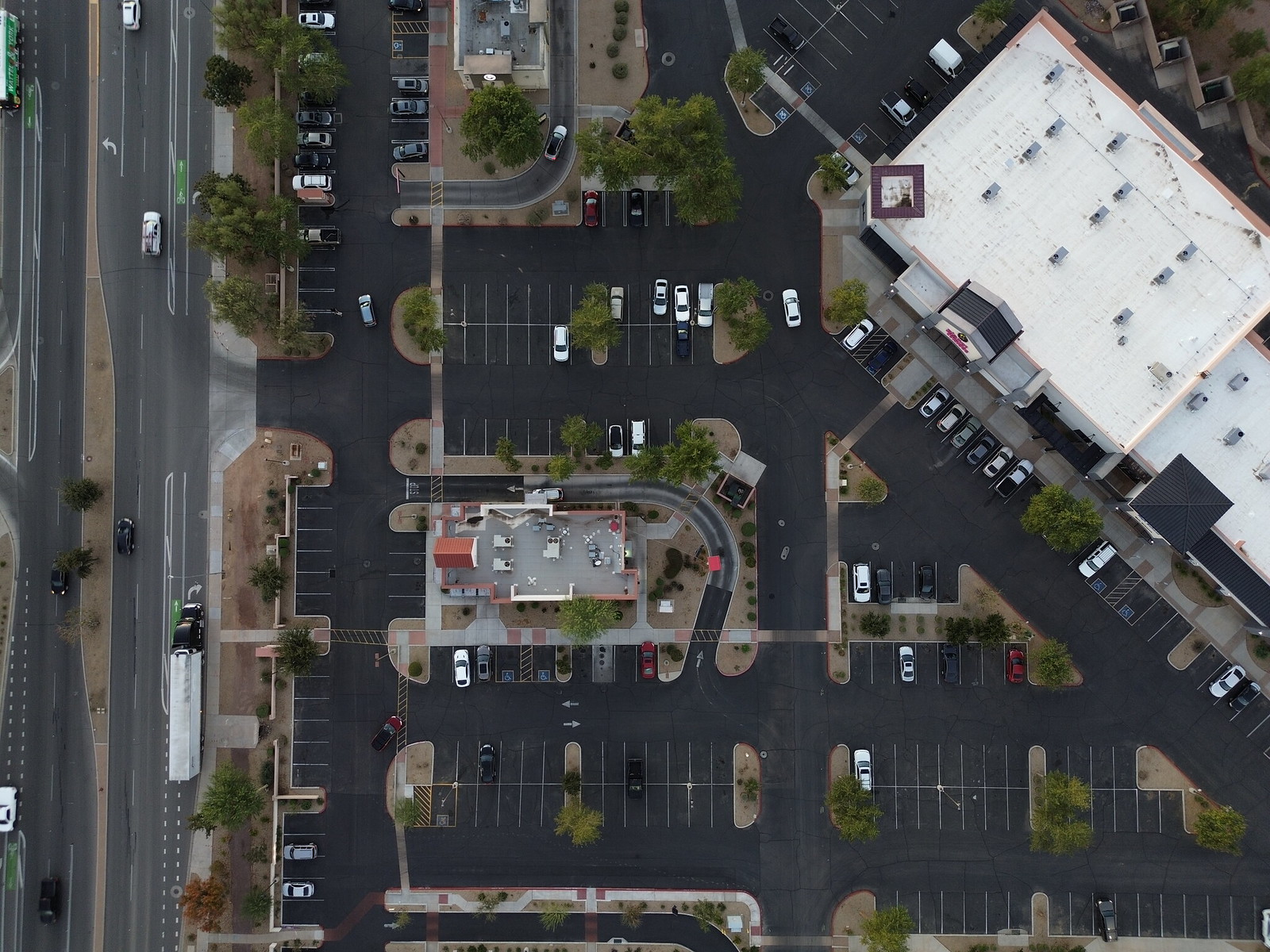This aerial photograph showcases a sprawling parking lot adjacent to a business establishment. To the left, a multi-lane highway with a median runs parallel to the lot, bustling with traffic that includes both passenger cars and 18-wheelers. The majority of the parking lot, composed of dark charcoal and black pavement, appears largely vacant with only a few scattered vehicles. In stark contrast, the highway's surface is of a lighter gray hue. Various clusters of trees punctuate the parking area at different intervals, adding a touch of greenery amidst the asphalt expanse. At the right side of the image stands a substantial building with a pristine white roof, fronted by several parked cars. This detailed overhead view captures the intricate layout and diverse elements of this commercial area.